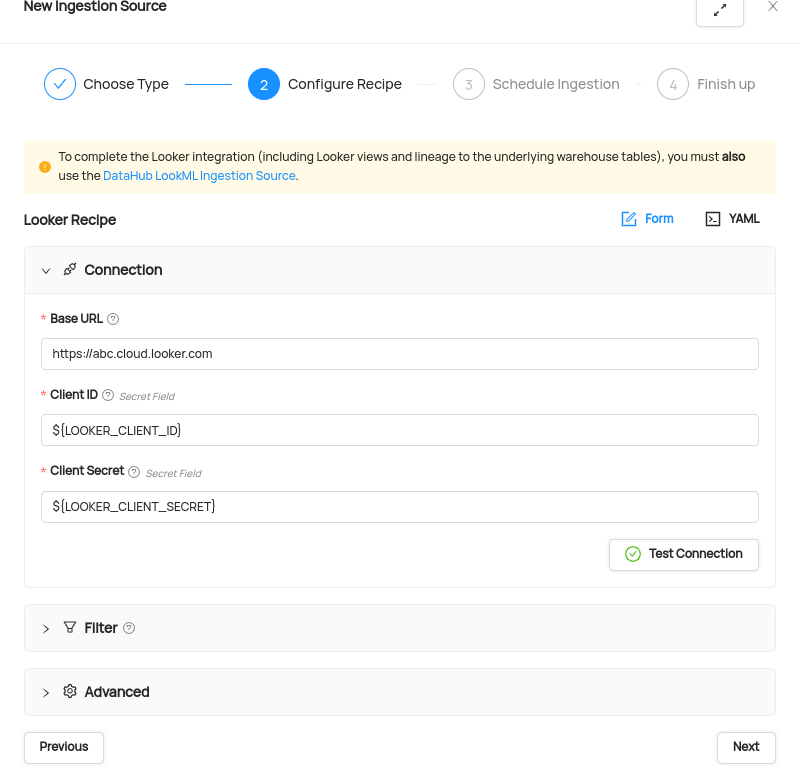A detailed and structured caption for the described image could be:

---

**Detailed Instructional Interface for Configuring a New Data Ingestion Source**

The image depicts an interface designed for setting up a new data ingestion source. Prominently at the top-left corner, the title "New Ingestion Source" is displayed in bold font. In the upper-right corner, there are icons for maximizing the window to full screen and for closing the window.

A thin gray line separates the top header from the main content area below, which guides the user through a four-step process. The steps include:

1. **Choose Type**: This step is marked with a blue checkmark, indicating completion.
2. **Configure Recipe**: The current step, highlighted with a blue circle containing the number 2.
3. **Schedule Ingestion**: A grayed-out step numbered 3, indicating the next step in the process.
4. **Finish Up**: The final step in the sequence.

Below these steps, a yellow informational box offers additional guidance. It reads: "To complete the Looker integration, including Looker Views and Lineage, to the underlying warehouse tables, you must also use the Data Hub LookML Ingestion Source." The phrase "Data Hub LookML Ingestion Source" is in blue and likely a clickable link.

The section titled **Looker Recipe** provides two format options, "Form" and "YAML," with "Form" currently selected. This section includes fields for:

- **Connection**: 
  - **Base URL**: Pre-filled with "HTTPS://abc.cloud.looker.com"
  - **Client ID**: Placeholder text "[Looker_Client_ID]"
  - **Client Secret**: Placeholder text "[Looker_Client_Secret]"

A button labeled "Test Connection" allows for testing the setup. Additional options include "Filter" and "Advanced Options," along with navigation buttons "Previous" and "Next" at the bottom of the page, facilitating smooth progression through the setup process.

---